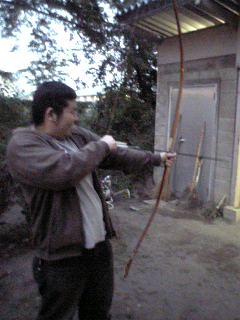The image is a photograph capturing a man with short brown hair and pale complexion in an outdoor setting, likely a backyard or similar area. He is actively pulling back a bow and arrow, preparing to shoot. The man is dressed in a gray or brown hoodie over a white t-shirt, with dark jeans. He stands on a dirt ground interspersed with patches of grass, surrounded by numerous weeds and shrubs. In the backdrop, there is a gray building with big tiles or bricks, featuring a metal awning, a door, and some lights hanging above it. The sky in the distance appears white and lit up, indicating daylight, and there's some tree cover visible far behind the scene.